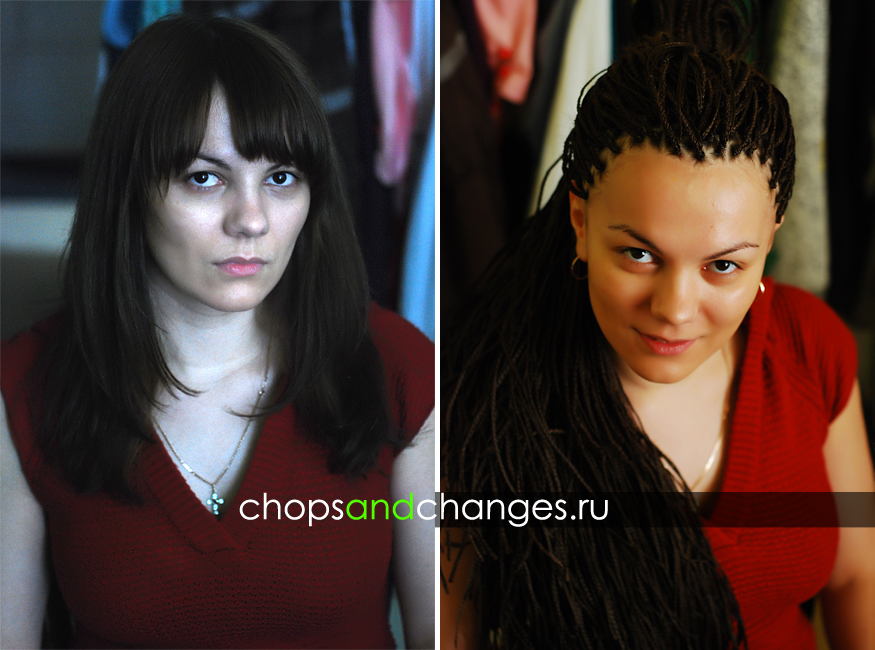The image is a landscape-oriented composite of two vertical color photographs placed side-by-side, each capturing a young woman in her 20s. Both women, framed against a background of out-of-focus clothing racks, look directly at the viewer. The woman on the left has short brown hair with bangs, dark black eyes, and a neutral expression with closed lips. Her attire includes a red knitted blouse and a cross necklace. In contrast, the woman on the right is African American, adorned with long braids cascading past her waistline, and sports a partial smile. She wears earrings and a red v-neck top. Dividing the two images is a black stripe featuring the URL "chopsandchanges.ru," with the word "and" highlighted in bright green. The piece combines photographic realism with elements of typography and graphic design.